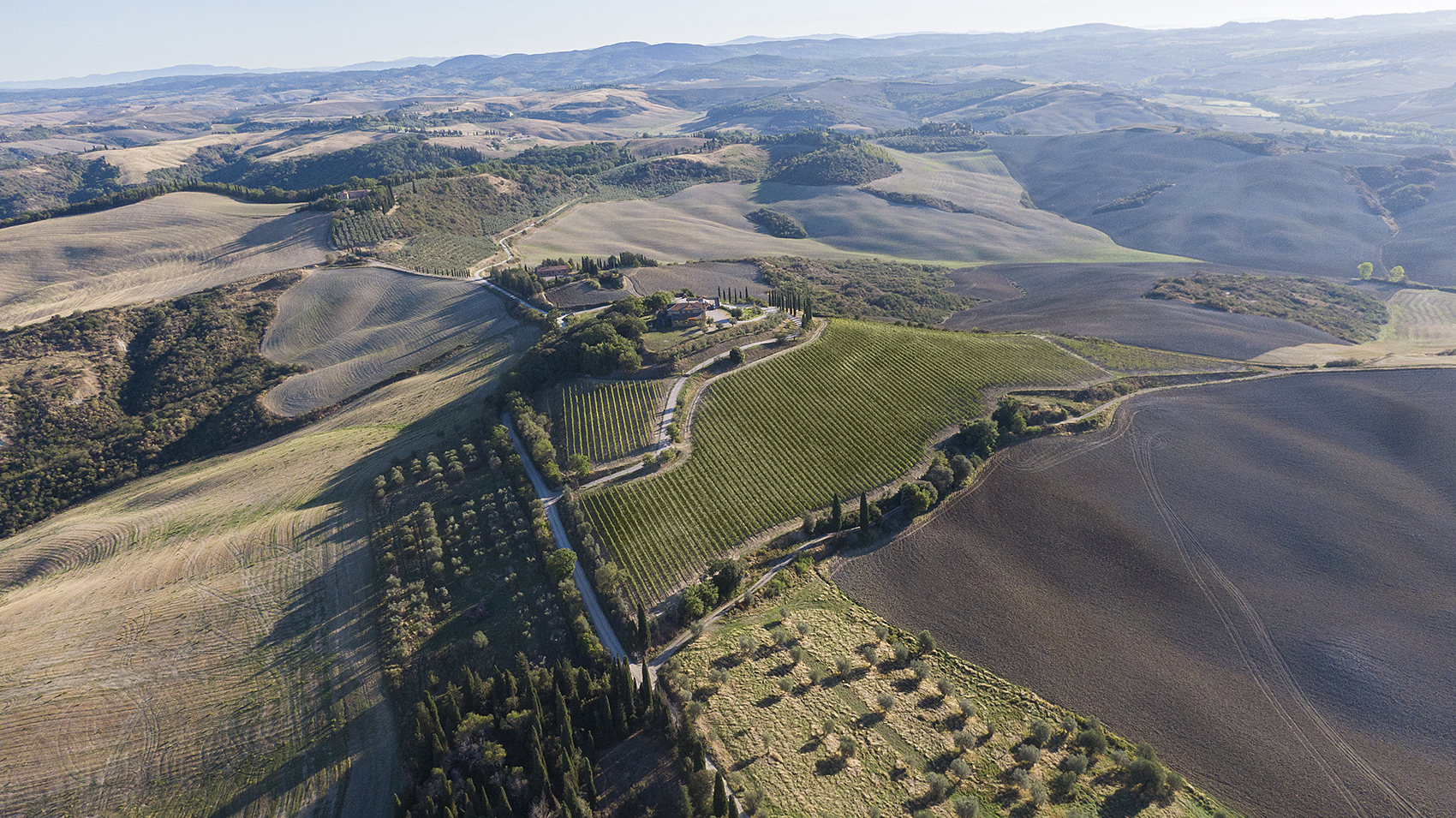An aerial photograph captures a hilly region meticulously divided into various cultivated zones and tillage areas. Directly beneath, a rocky terrain is interspersed with scrubby plants and a neatly arranged patch of evergreen trees in uniform rows. Adjacent to this, a lush hillside is adorned with rows of thriving green crops, separated by a winding roadway. A smaller section nearby features crops growing in distinctive ridged rows. In the midground, a residential area emerges, showcasing a house nestled among an assortment of trees. Stretching further into the distance, the landscape unfolds a mosaic of additional cultivated fields, painting a vivid picture of agricultural productivity against the natural undulations of the terrain.